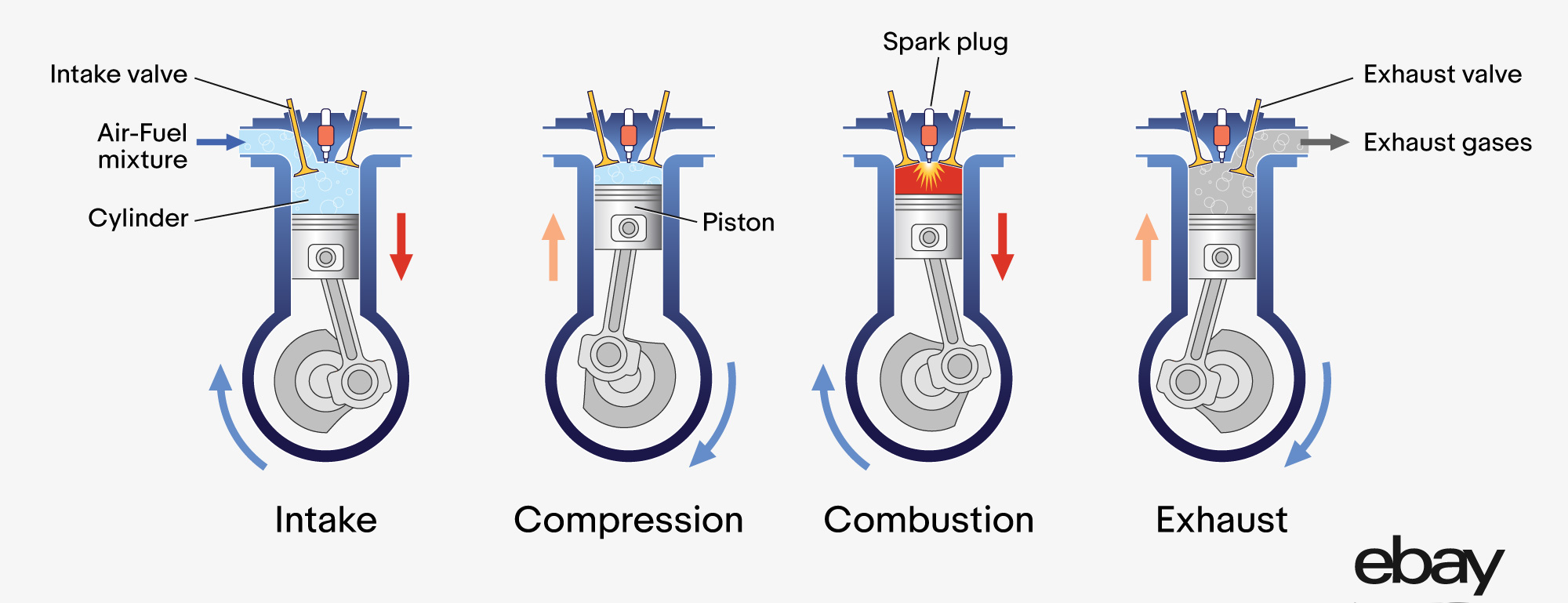The image is a detailed, hand-drawn diagram illustrating the four key stages of an internal combustion engine's operation, set against a gray background. From left to right, the stages are labeled as intake, compression, combustion, and exhaust. Each stage is depicted with distinct diagrams and labeled components. 
- In the intake stage, red and blue arrows indicate the air-fuel mixture entering through the intake valve into the blue cylinder.
- The compression stage shows the piston moving upward, compressing the mixture inside the cylinder.
- During combustion, the spark plug ignites the compressed mixture, causing the piston to move downward.
- In the exhaust stage, the exhaust valve opens, releasing exhaust gases through a designated tube. Throughout the diagrams, arrows illustrate the cyclical counterclockwise motion of the piston's mechanism.
In the bottom right corner, the eBay logo is prominently displayed in black.